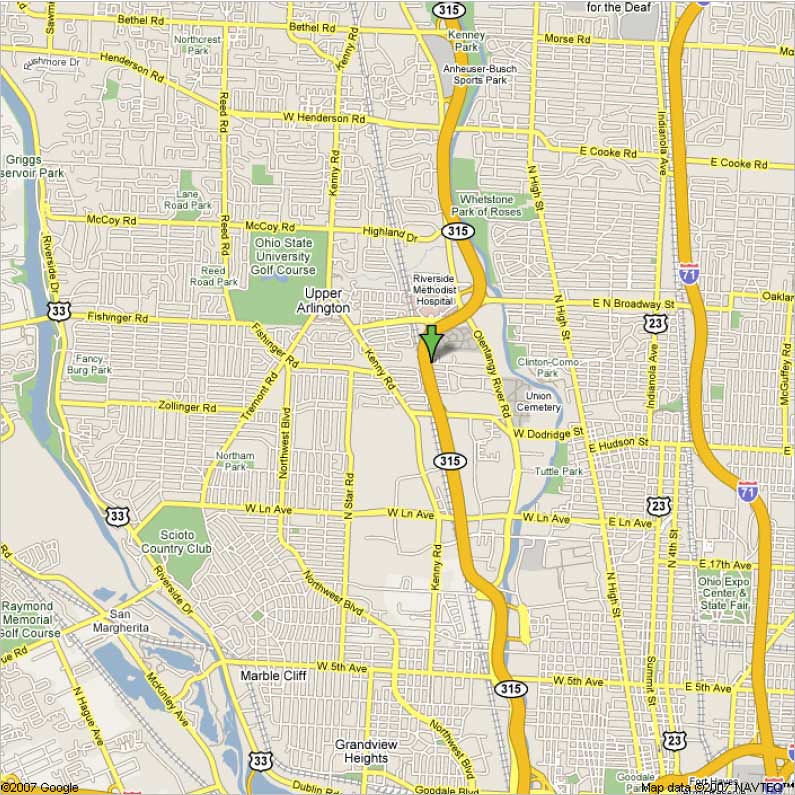This detailed map, sourced from a 2007 Atlas or Google Maps, includes data from 2007 Navteq (indicated by the marking "2007 Google" and "map data 2007 Navteq"). The map prominently features two main highways, identified as Route 315 and Route 71. A green arrow highlights a location on Route 315. Several landmarks are noticeable: to the left, the Ohio State University Golf Course is marked in green. Adjacent to Route 315 in the northern part, Kenney Park and Anheuser-Busch Sports Park are noted, while slightly further south, Whetstone Park of Roses is indicated.

Near the bottom of Route 71, the Ohio Expo Center and State Fair are labeled. An array of smaller, named and numbered streets crisscrosses the area, depicted in yellow lines. A river, depicted in blue, runs along the left side of the map, while Route 33, another significant route, runs north-south on the left side.